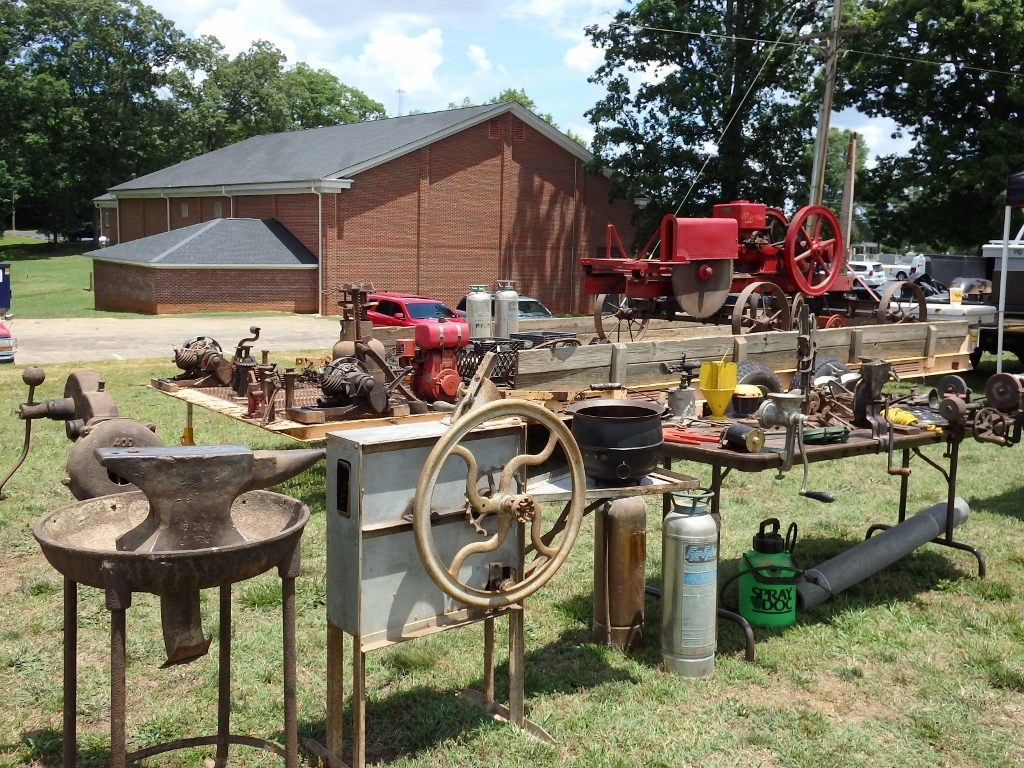This photograph depicts a yard area adjacent to a red brick home with a gray roof, likely in a historical or garage sale setting. On a grassy lawn, various metal yard tools and equipment are neatly displayed on tables and on the ground. Central to the scene is an old-fashioned, all-metal commercial mower or tractor, painted in red, with turning wheels and spokes, and topped with what appears to be a hand-crank engine. Nearby, there are several types of tanks, possibly for air, fuel, or insect repellent, including a gas tank and another unidentified tank, as well as a black cauldron and an anvil. Additional items include a clamp for woodworking, a tire, and other turning gadgets. A wooden trailer with an open back is also visible, laden with more metal tools and equipment. The backdrop features green trees under a blue sky with scattered white clouds, enhancing the impression of a quaint, nostalgic outdoor workspace.